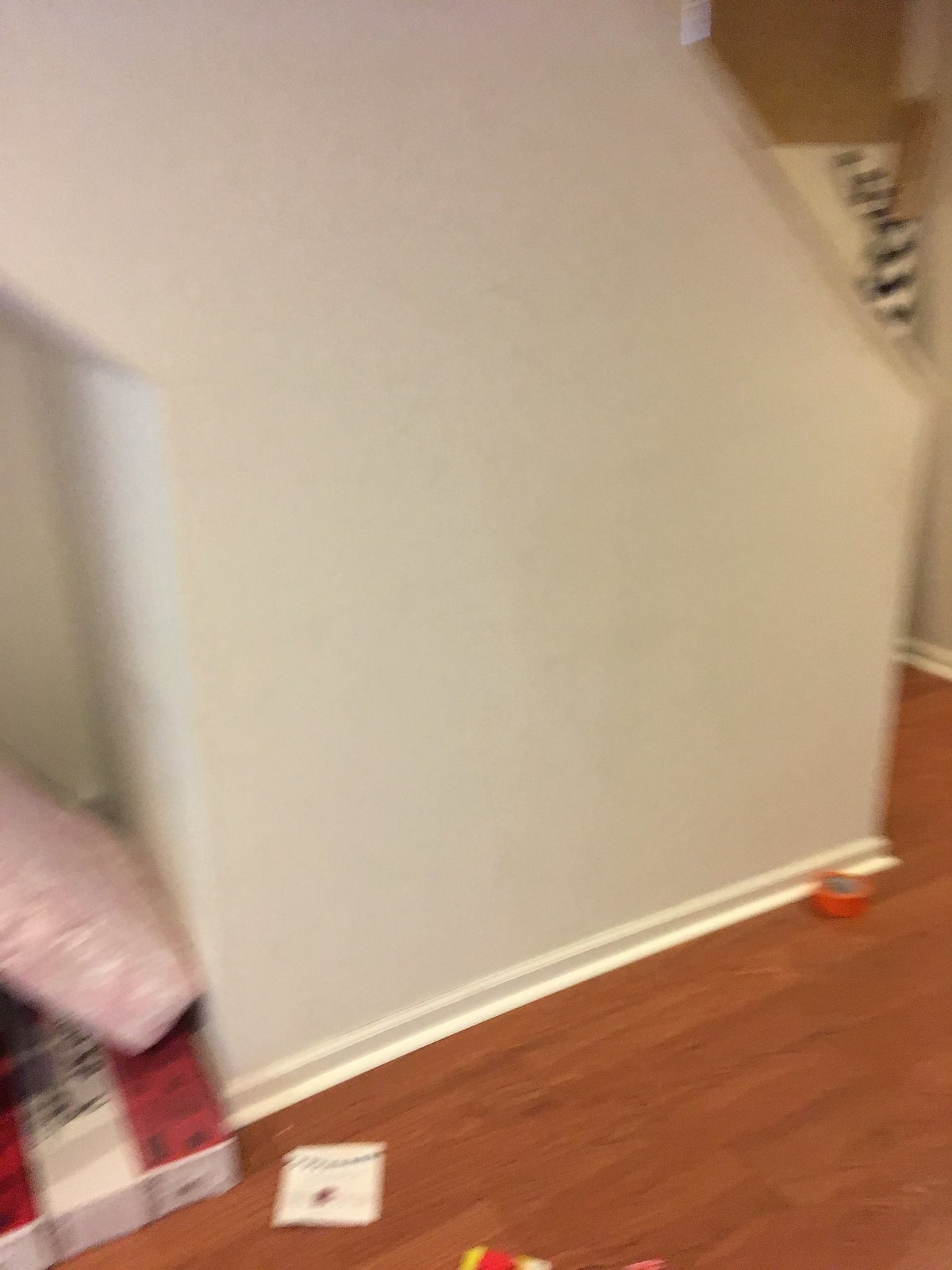The image, taken indoors, is somewhat blurry and out of focus, making specific details hard to discern. The scene features a light brown wooden floor, displaying darker brown wood grain patterns. The floor meets a white wall, accented by a white baseboard. On the left side of the image, there's a pinkish-colored box with some white areas, and its lid lies detached on the box's bottom. Inside the box, there's an object with red and white coloring. To the right of this box, on the floor, is a square-shaped white item with a black design at the top. Further along the floor against the wall, there's a circular orange object. Near the top right corner of the image, an outline of an object with black and white stripes can be seen.